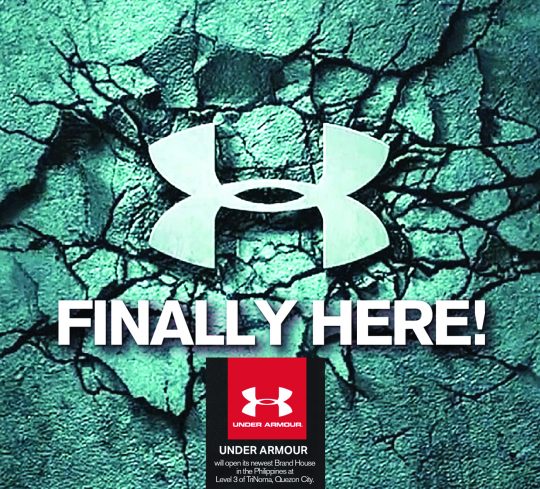The image features a textured background of cracked, dried-out clay with a grayish-blue hue. In the center, a deep indentation resembling an impact crater is prominently displayed. Within this indentation lies a bold symbol comprising a 'U' shape paired with an upside-down 'U' directly beneath it.

Above the symbol, bold white capitalized text exclaims "FINALLY HERE!" Below this text is a black rectangular section containing a red header where the same 'U' logo appears, this time accompanied by the phrase "UNDER ARMOR." Further down, within the black segment, the brand name "Under Armor" is mentioned again, along with some additional text that is too small to discern.